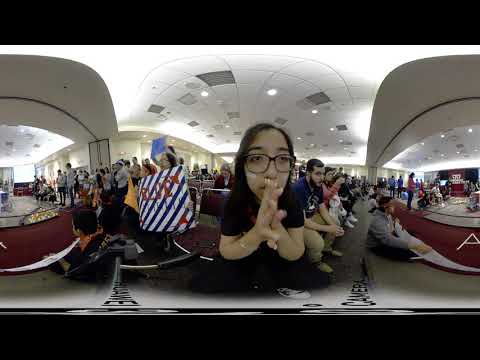In this vertical rectangle image, a large business-like area is depicted with a light gray ceiling, matching floor, and well-lit, very light tan walls. The spacious room is filled with people, many seated, suggesting a significant gathering. Dominating the center is a younger woman with straight, dark black hair and black-rimmed glasses. She wears a black short-sleeved top and appears deep in thought, her hands clasped in a prayer-like position covering her mouth. Behind her, the crowd extends, with several individuals holding signs. Notably, a person to her left holds a red and white striped sign turned away from the camera, while others have smaller blue and white signs. The setting, enhanced by the carpet's burgundy red hue, resembles an airport terminal, where people may be awaiting arrivals. The image also features horizontal black stripes at the top and bottom, possibly distorting the scene slightly.